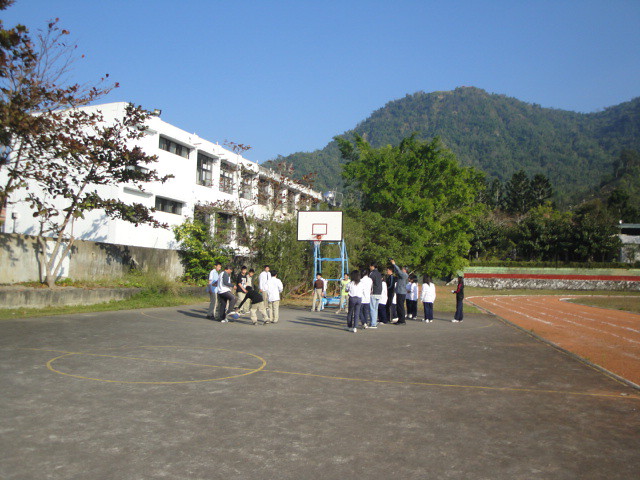The image captures a vibrant outdoor setting with a clear blue sky and a picturesque mountainous backdrop filled with lush green trees. In the foreground, the scene is dominated by what appears to be a school's exercise field. On the left side of the image, there is a stretched-out, white, two-story building, possibly a school, bordered by a red running track on the right. Central to the image is a grayish asphalt basketball court, which features a white basketball hoop and is surrounded by approximately 20 students, both boys and girls, engaged in activities around the hoop, perhaps picking teams or shooting hoops, indicative of a fall day as they are wearing jackets and pants. The entire scene is set against the majestic mountains, creating a dynamic contrast between the man-made elements and the natural environment.